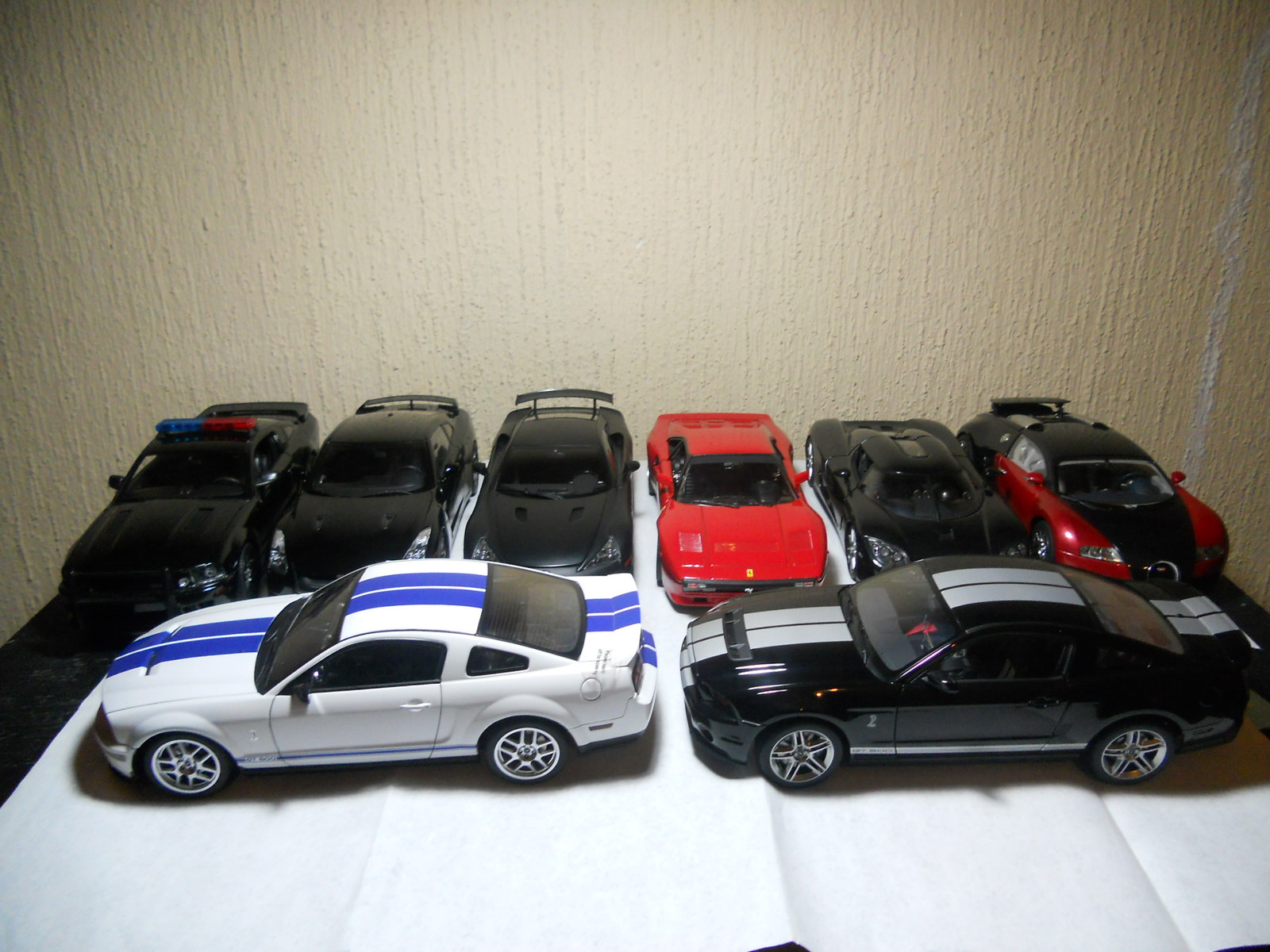This photograph showcases a vibrant collection of eight high-end model cars, meticulously detailed and scaled at 1:24 of their actual size. These premium metal models are arranged on a wooden table draped with a neatly spread out white cloth, casting a refined and sophisticated display. The setup is situated against a light brown, textured concrete wall that features subtle stripes, adding depth to the backdrop.

The cars are illuminated by a spotlight overhead, enhancing their shine and intricacies. In the foreground, two Ford Mustangs are prominently displayed facing sideways: one is a striking white model with bold blue racing stripes, while the other is a sleek black Mustang adorned with silver stripes.

The background row features a stylish assortment of six cars, all aligned facing forward. These include a black police cruiser, two additional black sports cars, a vibrant red Lamborghini, another sleek black vehicle, and a distinctive red and black sports car. The careful arrangement and thoughtful lighting create a captivating tableau that highlights the exquisite craftsmanship of these model cars.